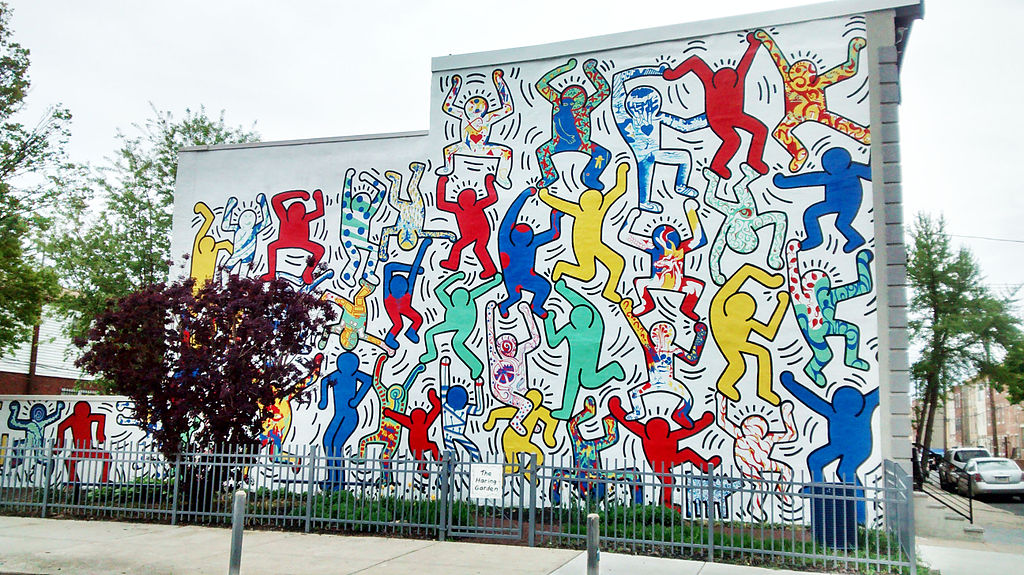In front of you is a cityscape captured in daylight, characterized by a clear white sky stretching across the background. Trees intermingle with buildings that create a busy urban environment. On the left side, a sidewalk is bordered by a light gray wrought iron fence, leading to a gate that opens into a green space known as 'The Healing Garden', indicated by a sign at the entrance. The fenced area features patches of green grass and some brown soil, providing a contrast to the surroundings. Dominating the scene is a flat-roofed building with two distinct heights; the front is taller than the back. Its wall is adorned with a vibrant mural showcasing abstract human figures engaged in various activities like jumping and dancing. These figures are depicted with simple round heads and without facial features, painted in a variety of colors including yellow, blue, red, green, and adorned with stripes and different designs. Black marks surround these figures, enhancing the sense of movement and energy in the artwork. To the right of the mural, a sidewalk with trees and parked cars continues to another building, creating a layered and dynamic urban setting.